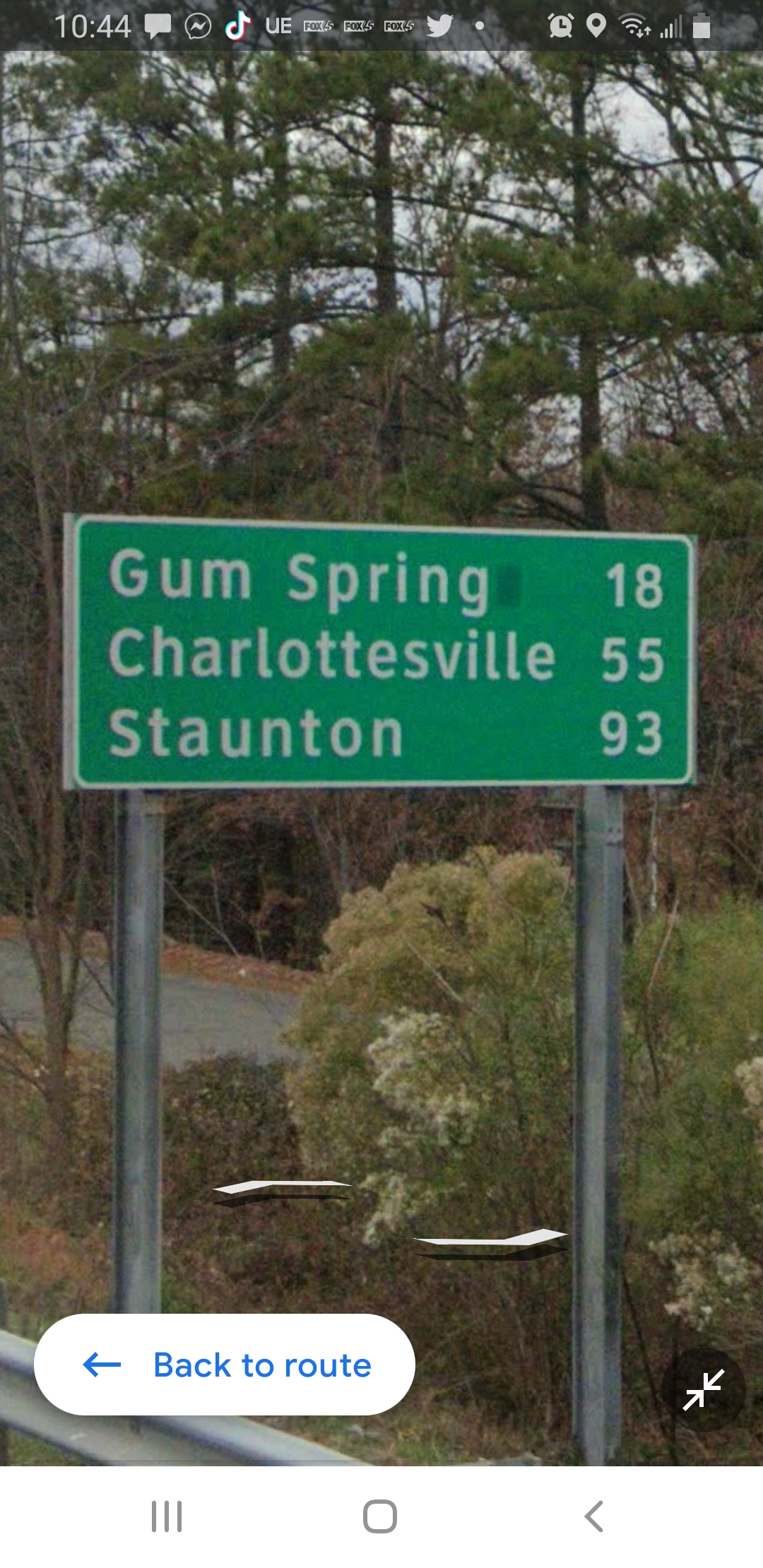This image, displayed on a cell phone screen, showcases a highway mileage sign situated at the edge of a road. The sign provides distances to nearby locations: Gumspring - 18 miles, Charlottesville - 55 miles, and Staunton - 93 miles. The backdrop features lush pine trees, adding a natural ambiance to the scene. At the top of the screen, various phone interface elements are visible, including the volume level, signal strength bar, battery level, current time (10:44), network indicator (UE), and the Twitter bird logo. The bottom of the screen features icons for expanding the image, as well as a thumbnail for returning to a previous view. This meticulous on-device screen captures an everyday roadside view framed by the digital trappings of modern mobile technology.